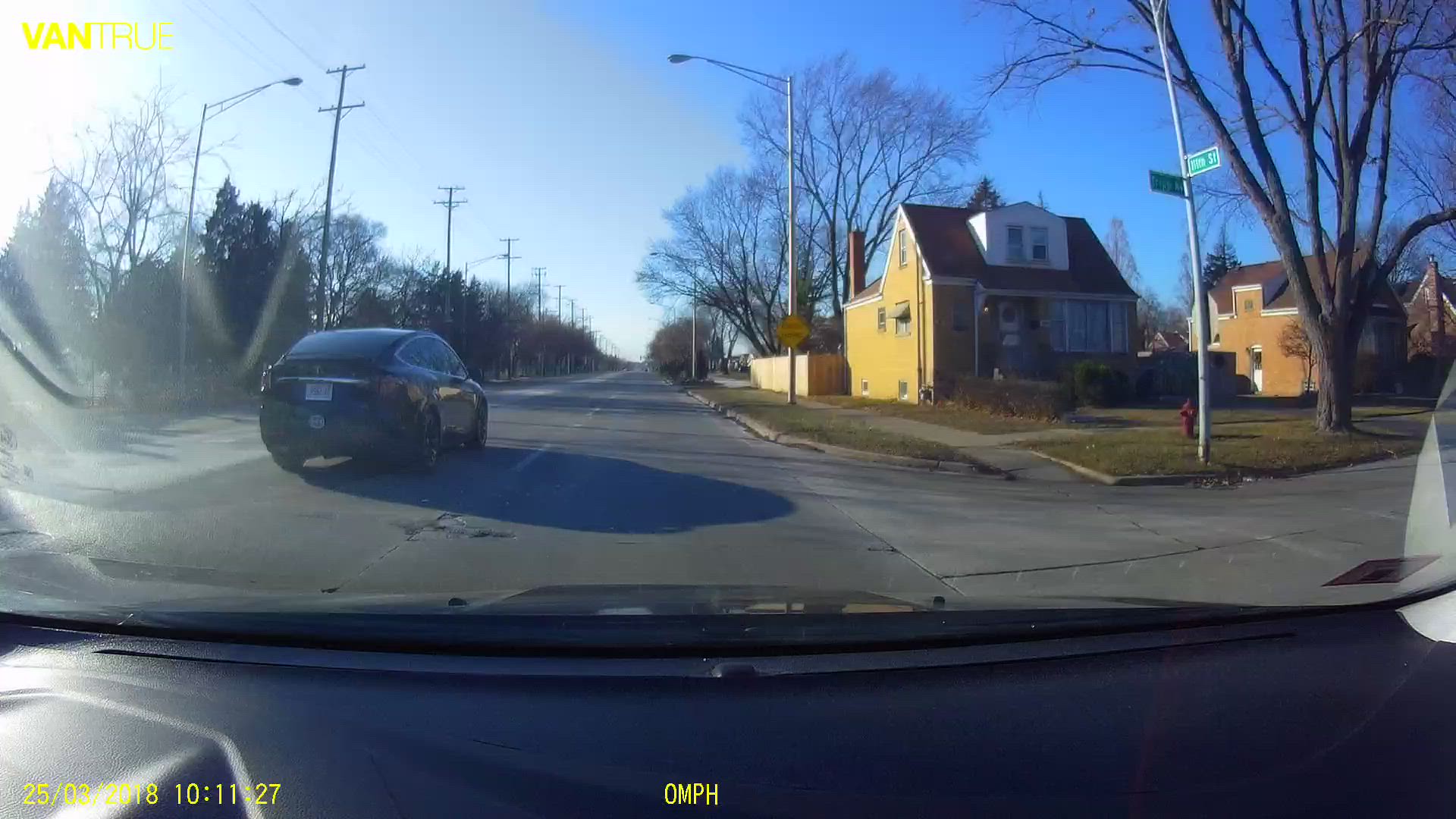This dashcam photograph, captured on March 25, 2018, at 10:11:27 from a Vantrue camera, showcases a suburban neighborhood street. Taken from inside a car, the black dashboard is visible along with the windshield glare. The image reveals a small two-lane street at an intersection with another street to the right, where houses with 1980s architecture—partially brick, partially vinyl siding—stand. The car is in the far right lane while a shiny, standard four-door car is seen in the left lane. A yellow house and a green residential street sign with two names appear to the right. The scene includes some road wear, like potholes, emphasizing the everyday nature of the suburban setting. All the dashcam's digital overlays, such as the date and brand name “Vantrue,” are displayed in yellow.